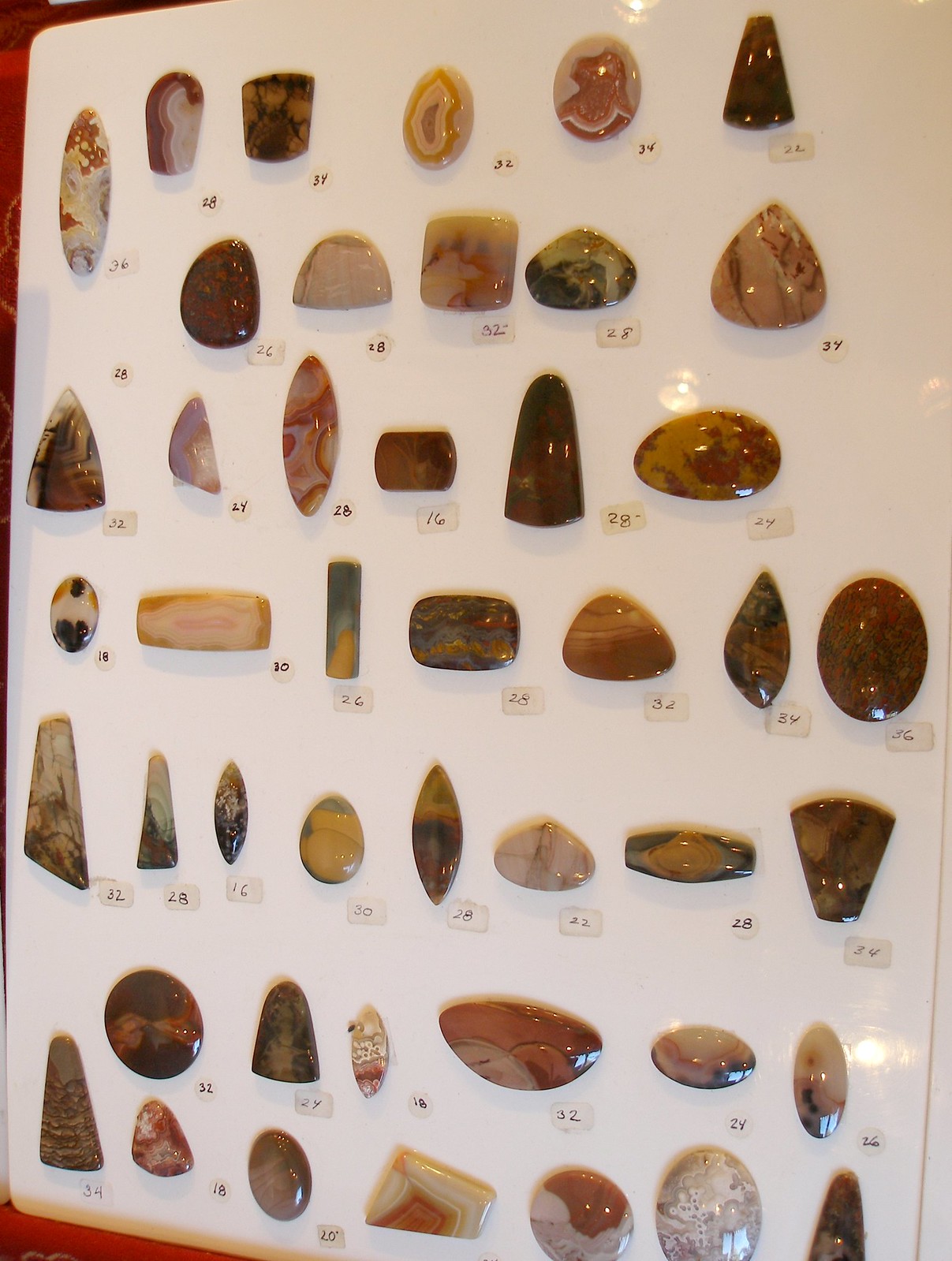This photograph captures an intricate display of polished stones and mineral samples, meticulously mounted on a plaque. The exhibit features an array of approximately 40 to 50 pieces, each labeled with a tiny number beneath it. The stones come in a variety of shapes including triangles, squares, ovals, rectangles, and circular forms, with some even resembling an ice pick. The color palette is diverse, featuring shades of brown, wine-colored red, light red, green, and even some translucent variations with hints of brown, black, and orange. Additionally, there are stones that are white and spotted. The stones' smooth, shiny surfaces suggest they have been carefully polished. The overall layout and labeling hint that this could be a display for potential buyers to select specific stones by their number. The photograph itself is void of any people or additional text, emphasizing the beauty and variety of the stones.